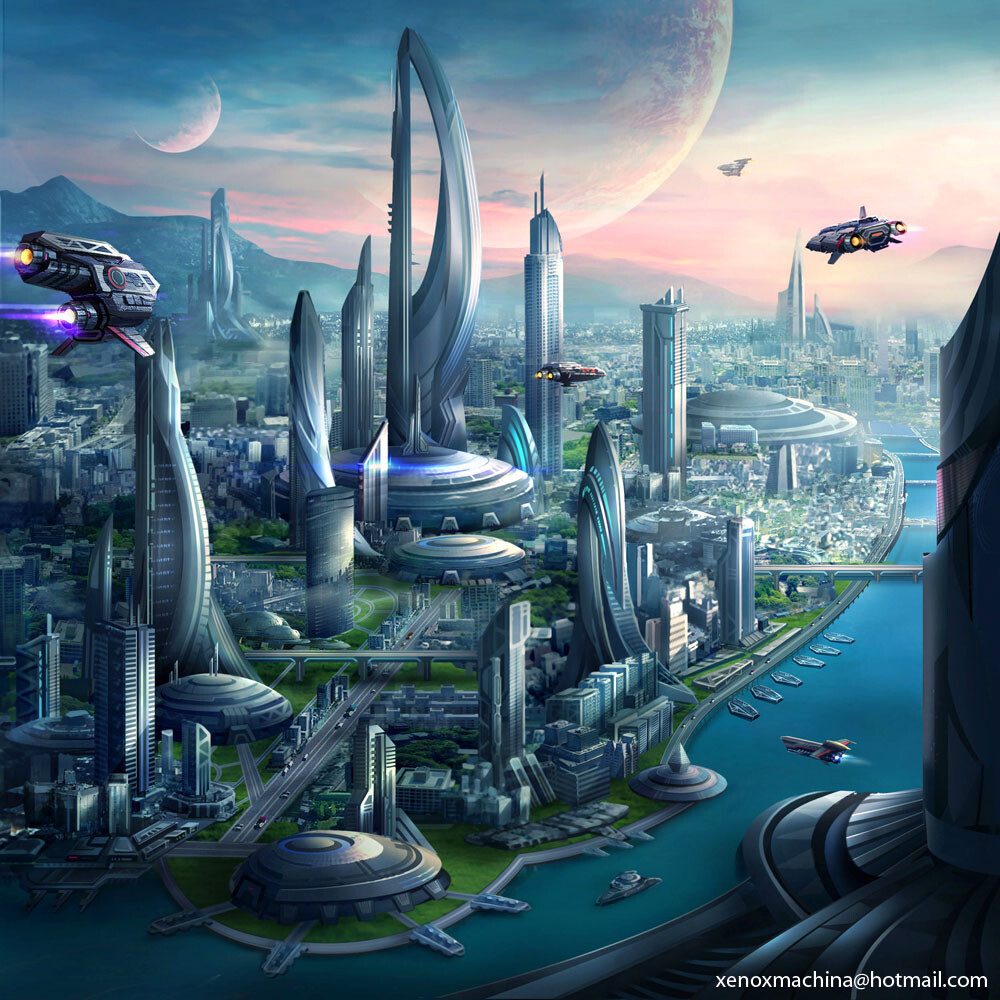This image is a highly detailed artist's rendition or a computer-generated depiction of a futuristic city that could easily be from a video game set in another world or on another planet. Viewed from an aerial perspective, the city sprawls along a shoreline with a river running through it. The skyline is dominated by many high-rise buildings, featuring tube-shaped and uniquely curved structures in a sleek gunmetal gray, unlike anything seen in contemporary architecture. 

Futuristic aircraft, emitting distinctive purple jet streams, are seen soaring through the skies, contributing to the otherworldly atmosphere. On the ground, there are fewer cars than one might expect in such a large city, further emphasizing the advanced, futuristic setting. Along the shore, various types of advanced-looking boats are pulled up, facing the water. 

In the distant sky, two large celestial bodies—resembling moons or possibly another planet—loom large, enhancing the otherworldly ambiance. The right-hand corner of the image bears a watermark in solid white font, reading "xenomachina at hotmail.com," likely indicating the artist's contact information.